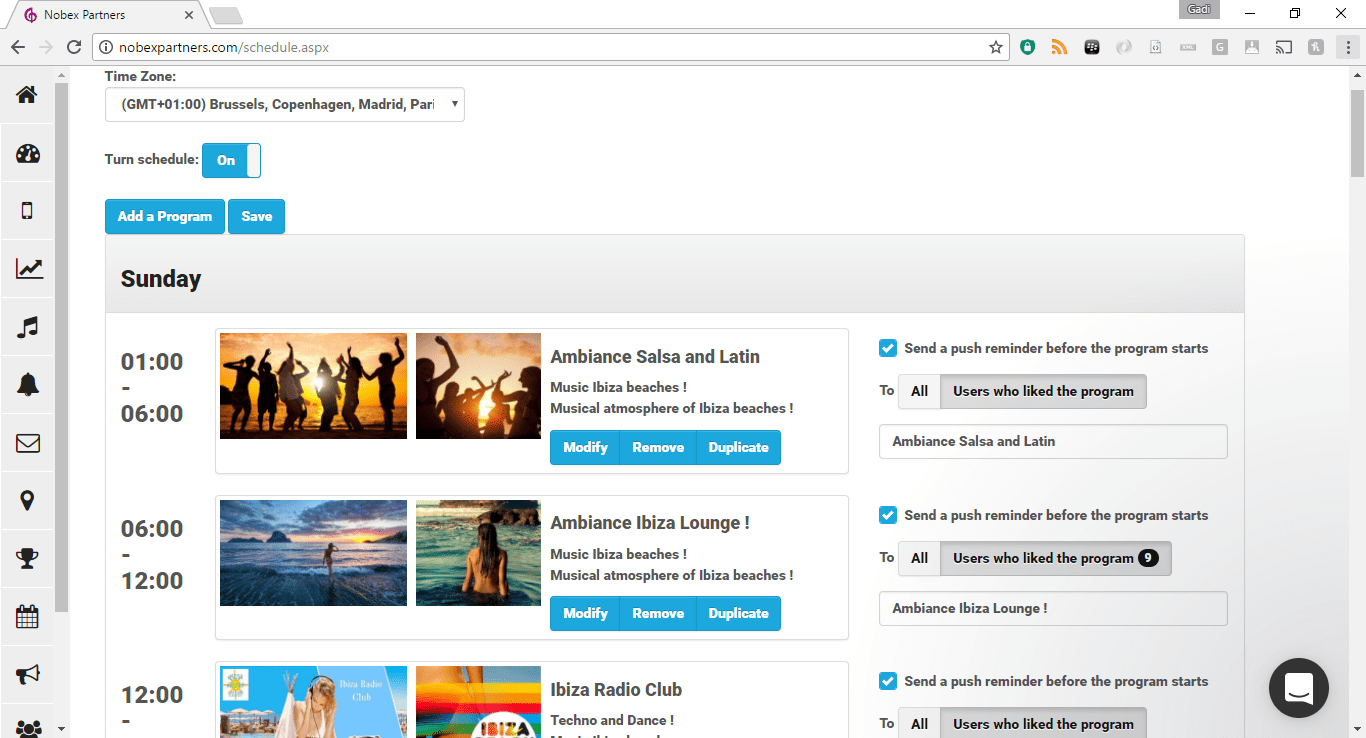Screenshot of Nobex Partners Schedule Page

The screenshot showcases the "schedule.aspx" page on nobexpartners.com, specifically highlighting various functionalities available on the Nobex Partners platform. The upper right corner features multiple buttons for different functions, excluding a battery indicator, suggesting this view is from a device like a laptop where power levels are not displayed. Additional shortcut buttons are found on the top right, culminating with a three-vertical-dots icon for more options.

The page specifies a time zone (Brussels, Copenhagen, Madrid, Paris) and includes dropdown menus and buttons for turning the schedule on or off, adding programs, and saving changes. The primary content focuses on a Sunday schedule, divided into segments showcasing different music programs and ambiance settings. 

From 1:00 to 6:00, the program includes "Ambiance, Salsa and Latin on the Beaches." Following that, "Ambiance, Ibiza Lounge Music" runs from 6:00 to 12:00, and starting at 12:00, "Ibiza Radio Club" is scheduled. Each program segment is accompanied by evocative photos of people dancing at sunset, frolicking on beaches, and enjoying the coastal environment, enhancing the visual appeal of the offerings.

The right side of the image presents options to send push reminders, all of which are enabled. This detailed set-up allows users to engage with complex reminder systems for scheduled activities. On the far left, a dock provides quick access to home, settings, music, alarm, email, calendar, and sound — creating a robust and multifaceted interface.

Overall, the page offers a comprehensive and user-friendly interface focused on music and entertainment programs scheduled for Sunday, enriched with beautiful imagery and functional options to enhance user experience. The design features a clean white background, adding to the clarity and ease of use.